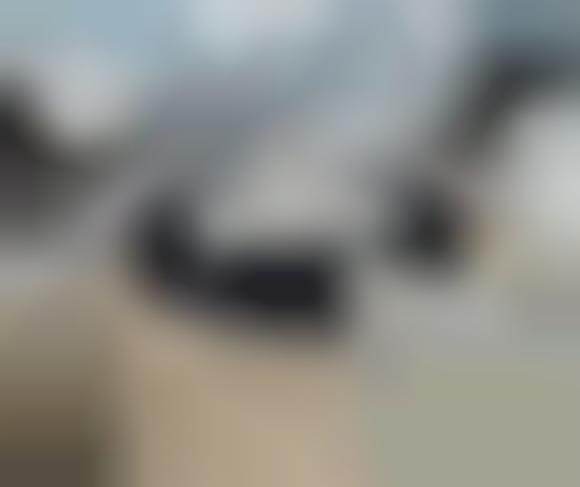This image captures an exquisitely luxurious lounge area, likely part of a high-end ski lodge perched atop a snowy mountain. The room is designed with a stark, dramatic aesthetic that combines comfort with sophistication. A large, clear window spans the upper portion of the photograph, offering breathtaking views of a snowy mountainscape, reinforcing the impression that this retreat is situated on the edge of a cliff. The lounge features black and white furnishings arranged around a stunning central fire pit. The seating includes white-framed chairs with black cushions and wicker sides, complemented by a sizable white couch with a black cushion and a white pillow.

At the heart of the room is a round fire pit, which serves as a focal point. This pit, encircled by shiny glass stones, features a striking crystal-like structure at its center, possibly a pseudo-fireplace designed to mimic flames. The fire pit's outer base is silver, with a line extending from its edge, housing potential controls. The light-colored carpeting adds a bright and vibrant touch, enhancing the overall ambiance of the lounge. This meticulously designed space epitomizes luxury, offering a serene retreat with panoramic views of the majestic snowy mountains.